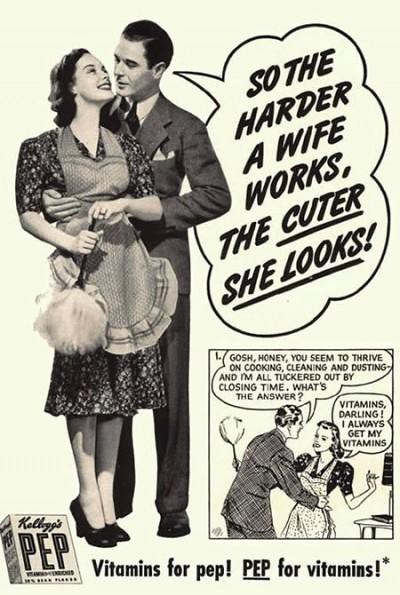This image features a vintage-style advertisement, reminiscent of a 1940s or 1950s newspaper or magazine clip. The central focus is a man and a woman dressed in period attire, capturing an old-timey cartoon aesthetic. The woman, situated on the left, is wearing a knee-length dress, a frilled apron, and black high heels, while holding a feather duster. She smiles as she looks up at the man, who stands to her right, dressed in a suit with a handkerchief in the pocket and black shoes. He is holding her by the waist and looking down at her, uttering the phrase in a speech bubble, "So the harder a wife works, the cuter she looks."

In the bottom right corner, the scene is mirrored in a more cartoonish style. Here, the same couple appears, with the man commenting, "Gosh honey, you seem to thrive on cooking, cleaning, and dusting and I'm all tuckered out by closing time. What's the answer?" The woman responds, "Vitamins darling. I always get my vitamins." Below this, there is a highlighted box of Kellogg's PEP Vitamins with the slogan, "Vitamins for PEP! PEP for vitamins."

The overall ad exudes a nostalgic vibe, effectively merging a modern recreation with classic, mid-20th century comic strip elements to promote Kellogg's PEP Vitamins.